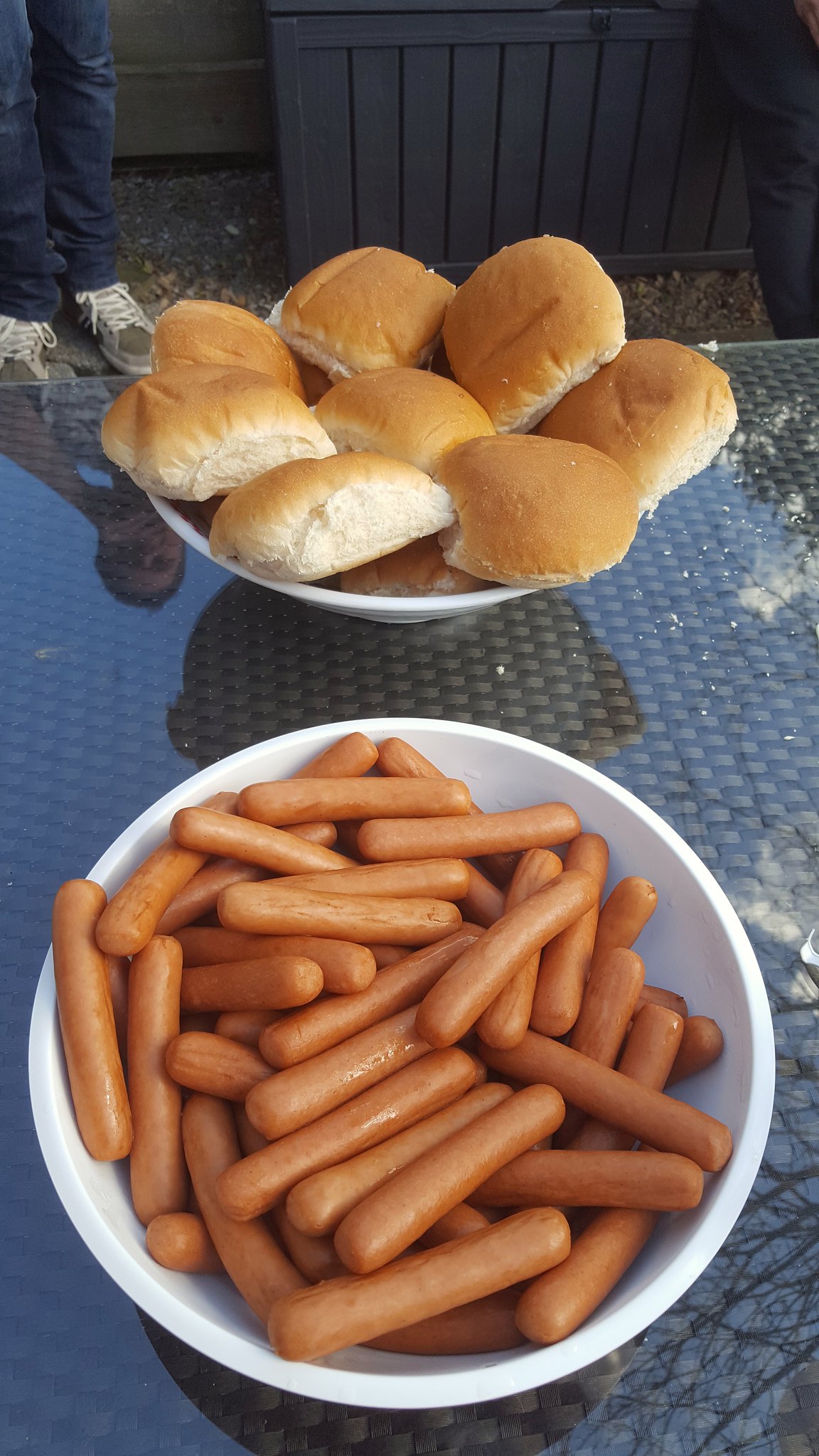This color photograph, taken outdoors in portrait mode, captures a detailed scene centered around a glass-topped table with a woven texture beneath. On the table, there are two large, white ceramic bowls. The bowl in the foreground is heaped with at least 30 hot dogs, jumbled together without any condiments or buns. The bowl behind it contains approximately a dozen brownish hamburger buns, contrasting with the hot dogs. Reflecting off the shiny glass surface of the table, you can see a blue sky with clouds and bare tree branches. There is also a reflection of a person's head with their hand near their mouth. Behind the table, you spot a person in gray sneakers with white laces and dark blue jeans, extending slightly past the knee. In the far right corner, another individual leans against a wall, also wearing jeans. The setting suggests a casual backyard gathering with minimal detail in the background, apart from a glimpse of a black wooden fence.